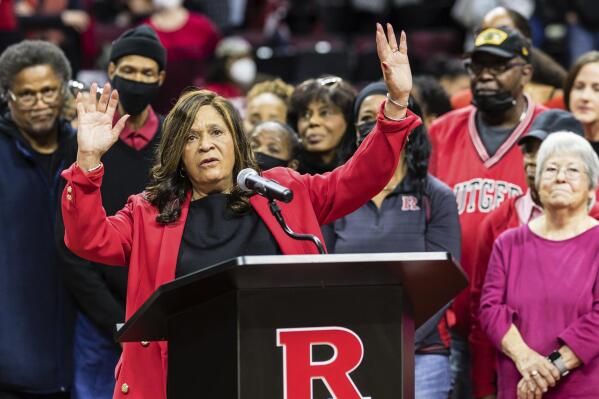In the image, a distinguished older Black woman stands confidently at a black podium adorned with a prominent red "R" emblem, representing Rutgers University. She wears a striking red suit jacket over a black blouse, her hands raised expressively beside her head. Her long hair flows to the top of her chest as she speaks into the microphone. Surrounding her at the podium are diverse individuals, predominantly Black men and women, interspersed with one white woman sporting granny glasses and a purple top. Among the group, one man stands out with a Rutgers jersey, and another with a black knit cap and face mask. The gathered figures are all focused intently on something in the distance, lending a sense of gravitas and attention to the woman's address.